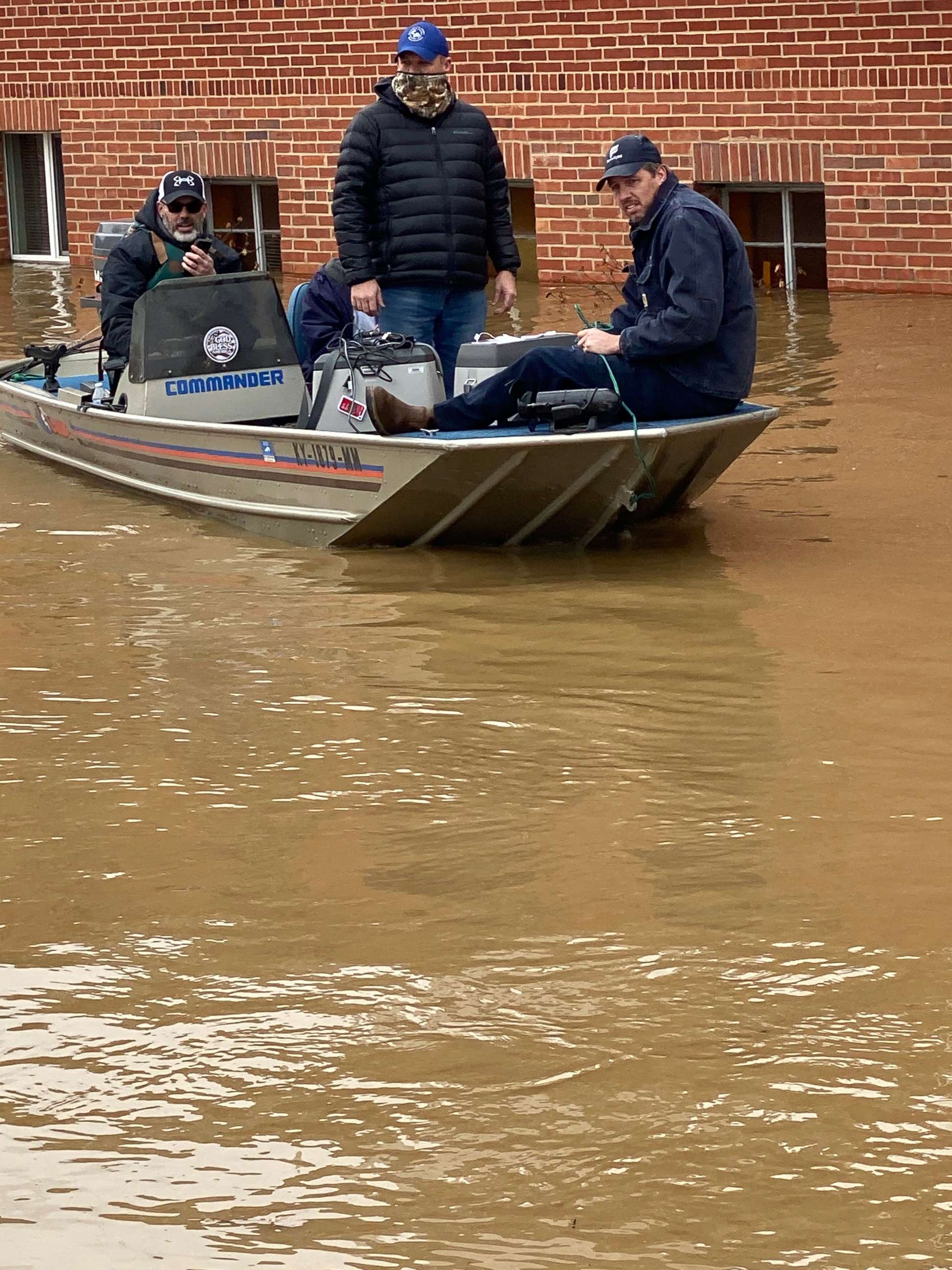The image depicts a small rescue boat navigating through murky brown floodwaters in a heavily flooded area during the daytime. The background features a brick building with water levels reaching up to its windows, indicating severe flooding. Inside the boat, which is a small metal craft marked "Commander," are four fair-skinned men, all dressed for cold weather in jackets and caps. One man, sporting a bubble jacket, stands in the middle, while two others are seated at the front and back. The man at the back, who has a gray beard, glasses, and a black-and-white hat, appears to be talking on a phone or radio, possibly coordinating the rescue operation. All the men are wearing similar hats, suggesting they might be part of a uniformed team. They seem to be surveying the flooded area for survivors.